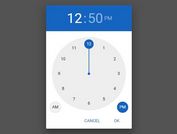The image features a rectangular frame with a prominent gray border that gradually transitions from nearly black at the top to a lighter gray towards the bottom. The top and bottom sections of the border are thin, while the sides are significantly wider. 

Inside the frame, there is a triangular-shaped box oriented vertically. The top part of this box is bordered in dark blue, containing the text "12:50 PM" in white letters. Below this, a circular clock face is displayed in gray. The clock shows numbers from 1 to 12, with an additional blue circle around the number 12 connected by a blue line to the center of the clockface.

On the left side of the clock, there's a gray circle marked "AM," while on the right side, there's another gray circle marked "PM." Additionally, a blue circle on the right side highlights "PM."

At the bottom of the frame, two buttons are situated—on the left, the button reads "CANCEL" in gray capital letters, and on the right, the button reads "OKAY" in matching gray capital letters.

This image appears to be a screenshot of a digital time-setting interface.